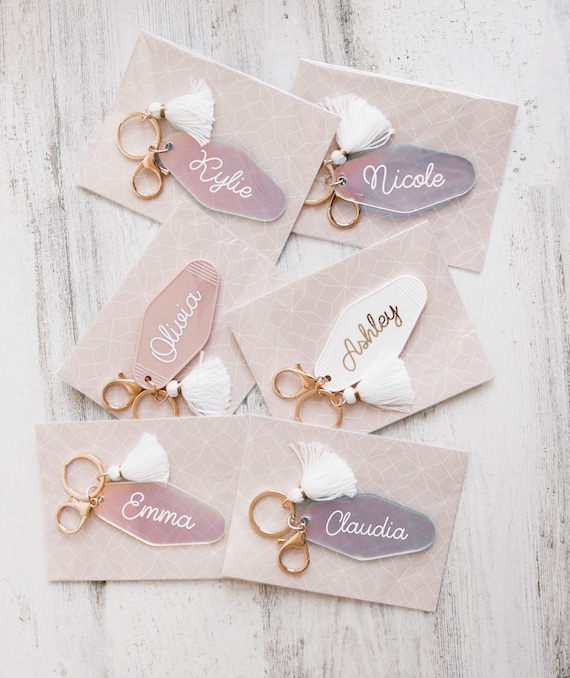The image displays an arrangement of six keychains, neatly placed in two rows of three on a light pink surface adorned with gray streaks. Each keychain is rectangular and features a pinkish-purple color with white geometric patterns. Attached to each keychain is a golden ring and a golden lobster clasp, from which hangs a white tassel and a small nameplate. The names on the keychains include Kylie, Nicole, Olivia, Emma, and Claudia, monogrammed in white. One keychain stands out; labeled with the name Ashley, it features a gold monogram on a white background. This distinct detail suggests it might be a special gift for the maid of honor, while the other keychains are likely for bridesmaids.